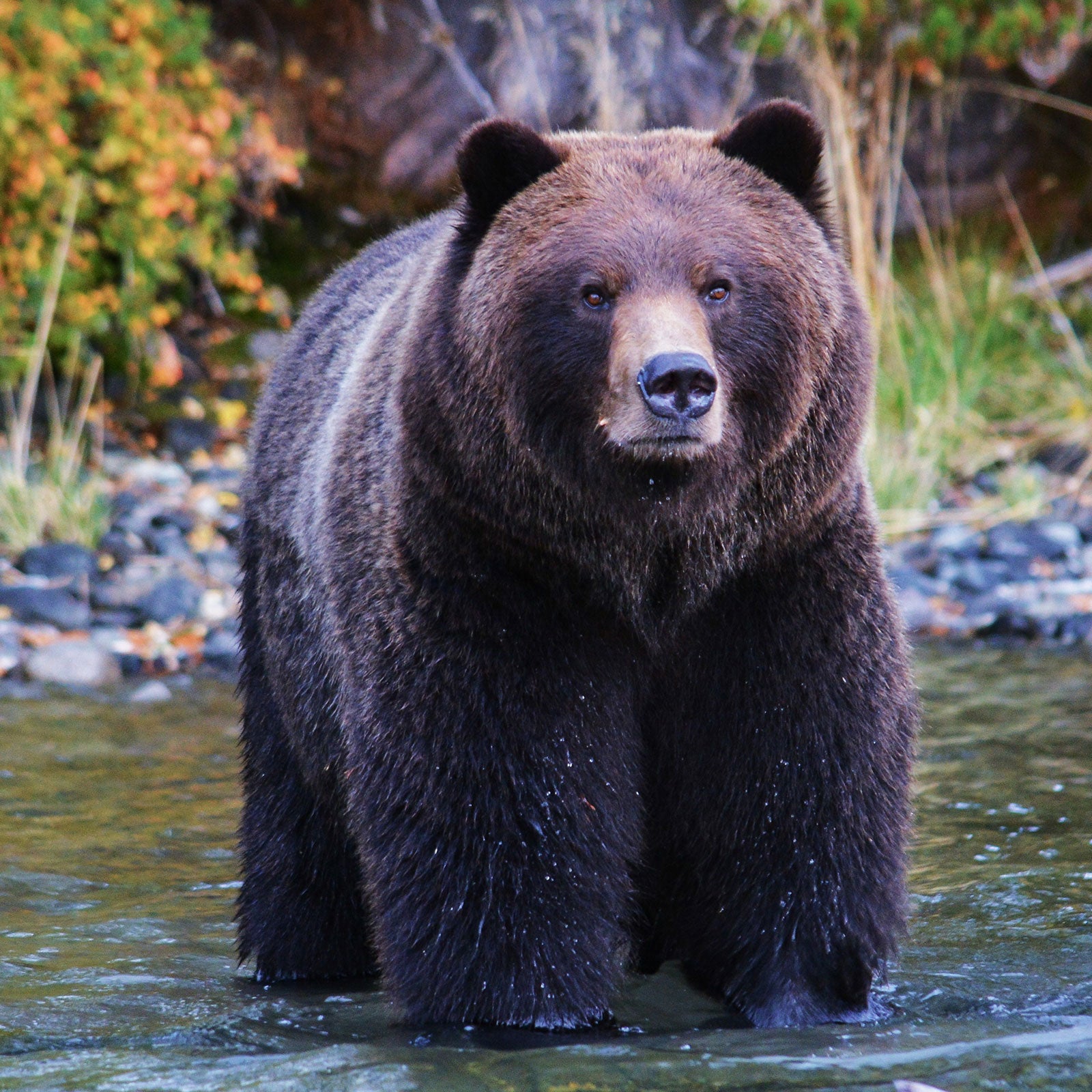In a square, daytime photograph, a large, well-fed brown bear stands in the middle of a shallow, dark gray stream, its fluffy, rounded legs partially submerged in the clear, wavy water. The bear appears calm, gazing directly at the camera with small, brown eyes contrasting its large, round face. Its light tan muzzle and black nose stand out against the darker brown fur of its head, which is almost black in parts, particularly around its perked ears that hint at some silver on his back. The shallow water, reflecting a mix of brownish and greenish tints, splashes slightly up on the bear's fur as it walks. In the background, a blurred mix of greenery, possibly bushes with orange flowers, and orange-tinged leaves cover the rocky shoreline, suggesting a fall setting.